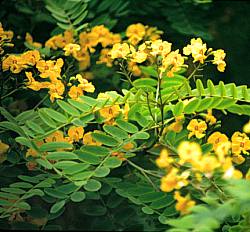This image depicts a flowering plant with distinct fern-like leaves and vibrant yellow flowers. The plant features elongated stems adorned with oval, fern-like leaves that are arranged in parallel rows on either side. Interspersed among the foliage are numerous small flowers, each with four or five wavy petals and an orangish spot at the center, reminiscent of snapdragons. These flowers are primarily concentrated in the central area of the image, stretching horizontally from left to right, while the top and bottom sections showcase only the verdant leaves. The photo is a square close-up with a noticeably low resolution, contributing to a slightly blurry or pixelated appearance. The foreground foliage appears lighter, contrasting with the darker green leaves and the dark, out-of-focus background, creating a vibrant tapestry of green and yellow hues.